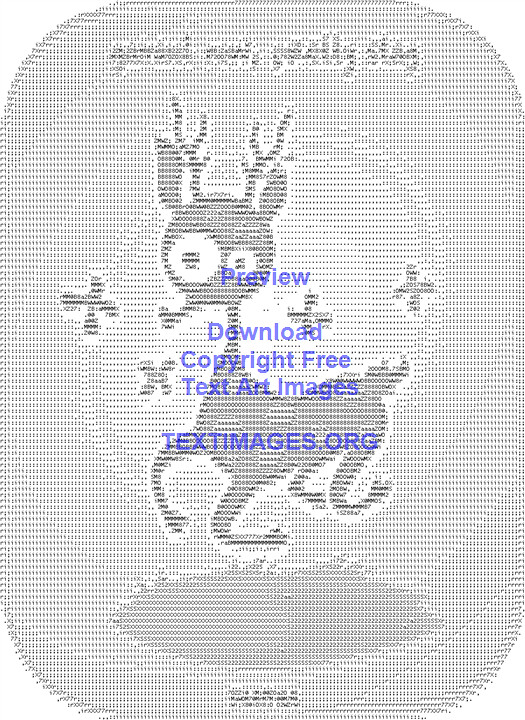The image is a detailed, computer-generated black and white graphic character, depicting a reindeer with a slightly gray tone. The reindeer is creatively rendered using a variety of letters, numbers, and symbols, such as zeros, 20s, and Zs. The character appears to be galloping with bent legs and is seemingly in mid-air, giving the impression of flying. Its distinctive features include a thin nose, uneven antlers— with the left one taller— and asymmetrical eyes, with the left eye being larger. Surrounding the reindeer are four-leaf clover-like shapes and possibly starry figures. The image also displays its shadow on the ground, portrayed as an oblong or rounded shape. At the top of the image, there is text written in blue or purple that reads "PREVIEW, DOWNLOAD, COPYRIGHT FREE, TEXT ART IMAGES, textimages.org" in all caps.